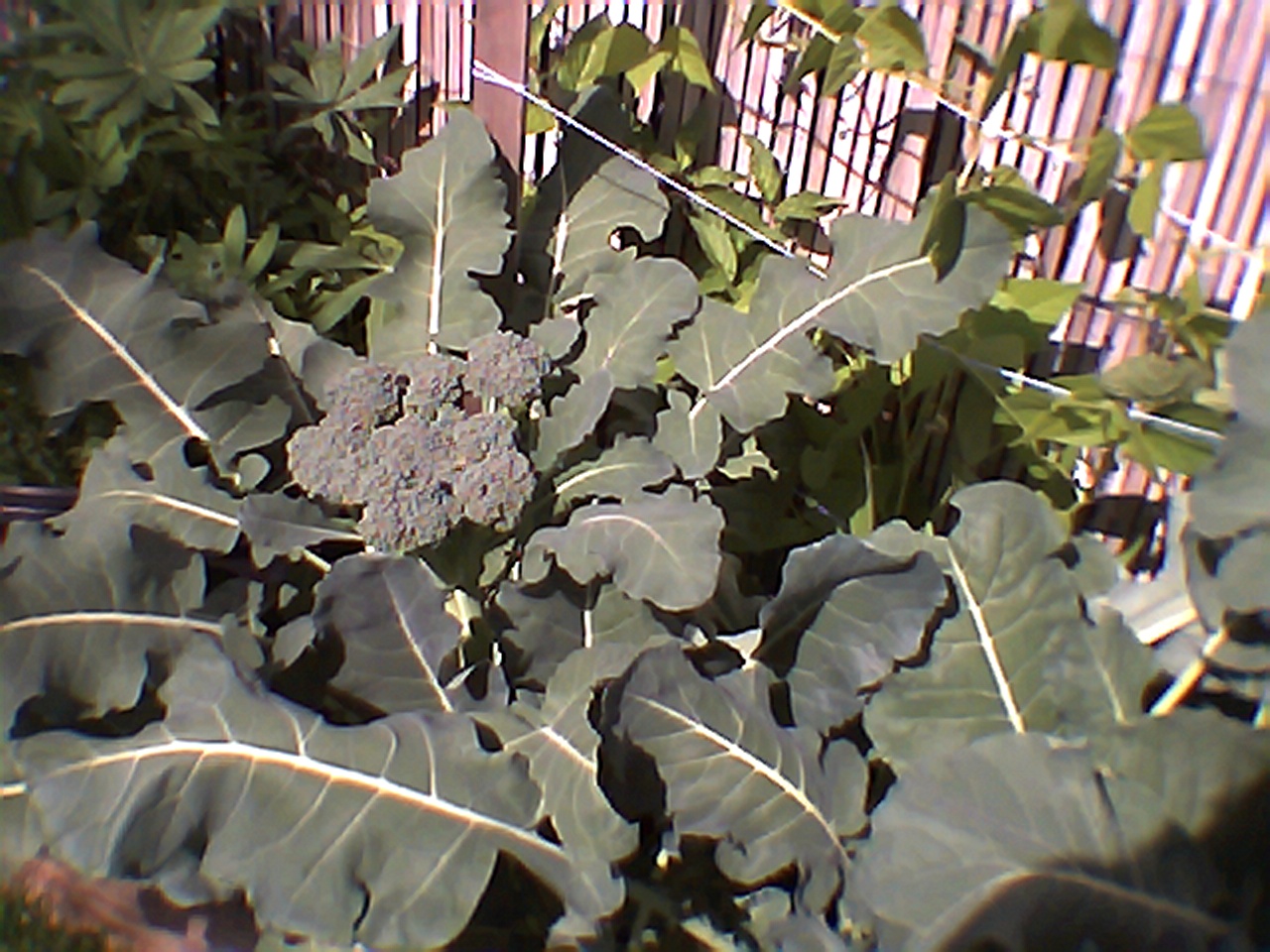The photograph, taken in landscape format with a low resolution, depicts a vibrant outdoor garden setting. The central subject is a small head of broccoli, positioned slightly to the left. It is sunlit, accentuating the plant's characteristic thick, grayish-green leaves with white veins. The broccoli head appears a bit loose, with spaces between the stalks, but the individual flowers remain tight and haven't started to bloom. Surrounding this main plant, more broccoli plants and leaves can be seen, particularly in the bottom right corner. 

Behind the broccoli, there is a notable gardening setup with a wooden stake, connected by white string to another post or structure off-frame. This string likely supports other plants, such as green beans or tomatoes, with vining green leaves growing upwards. In the background, a slat wood fence painted in burgundy and white stretches across the upper part of the image, adding a rustic touch to the garden scene.